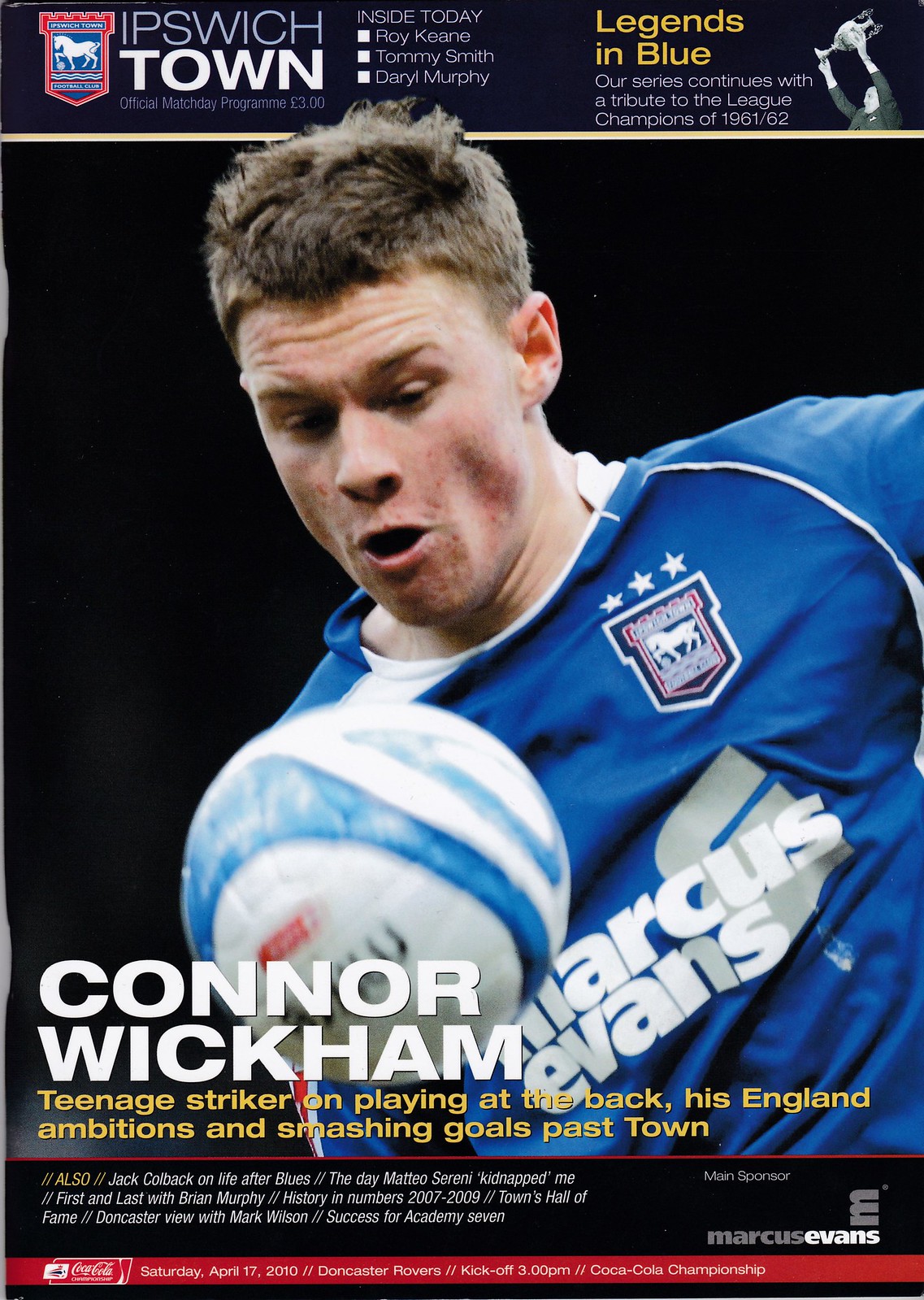The cover of the Ipswich Town magazine, which serves as the official match day program priced at $3, prominently features Connor Wickham in a blue soccer outfit, his upper body shown with his eyes focused downward at a large ball behind his name. At the top left of the cover, in grey uppercase font, the title "Ipswich" is displayed, followed by "Town" in large bold white caps. Also at the top, "Inside Today" highlights articles on soccer icons Roy Keane, Tommy Smith, and Daryl Murphy. A special tribute continues in blue and yellow font, honoring the league champions of 1961-62 under the title "Legends," accompanied by an image of a person lifting a trophy. At the bottom left, in white all caps, it says "Connor Wickham," and a yellow caption describes him as a "Teenage Striker" discussing his England ambitions and goal-scoring prowess. The bottom of the cover also provides match day details in a red bar, including the date Saturday, April 17, 2010, the opponent Doncaster Rovers, the kickoff time at 3, and noting the game is part of the Coca-Cola Championship.